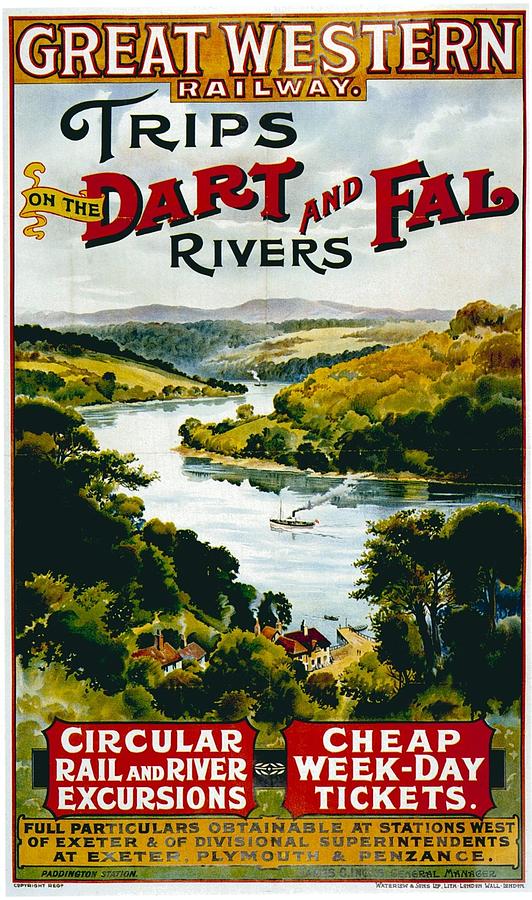This vintage promotional poster for the Great Western Railway advertises exciting trips on the Dart and Fall Rivers. At the top, a gold border proudly features the text "Great Western Railway" with "Trips on the Dart and Fall Rivers" written beneath a cloudy skyline. The centerpiece is a beautifully hand-painted image of a river meandering through lush greens and yellows, flanked by trees and scenic landscapes. On the river, a steamboat churns calmly, sending up a trail of steam. By its side, a port with quaint houses and a dock can be seen, capturing a serene yet appealing view. 

The lower part of the poster features two text boxes reminiscent of tickets: one in red announcing “Circular Rail and River Excursions Cheap Weekday Tickets,” and a yellow one below stating, “Full particulars obtainable at stations west of Exeter, and of Divisional Superintendents at Exeter, Plymouth, and Penzance.” The artwork uses an earthy color palette of greens, browns, yellows, and beiges, contributing to its nostalgic appeal. In the distant horizon, the silhouette of mountains adds to the picturesque scene, making this poster an enticing invitation to a scenic and adventurous rail and river excursion.